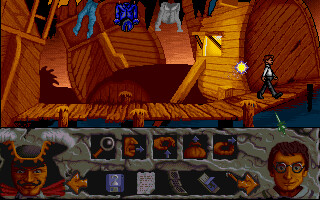This small rectangular image is a screenshot from a basic video game, showcasing a scene set inside a boat. Dominating the center of the screen is a wooden walkway, composed of textured wooden boards and flanked by wooden poles on either side, stretching horizontally from the left to the right. The left side of the walkway appears to connect to the interior of a boat, while the right side seems to lead to the entrance of another section of the boat. Keeping with the nautical theme, a clothesline is strung across the top of the image, attached to the tops of the boat's structures on each side. In the bottom-left corner of the screen, a detailed depiction of a pirate can be seen, while the bottom-right corner features an image of a nerdy-looking man with round glasses. An action bar is prominently displayed at the center bottom of the screen, likely containing various in-game options for interaction.